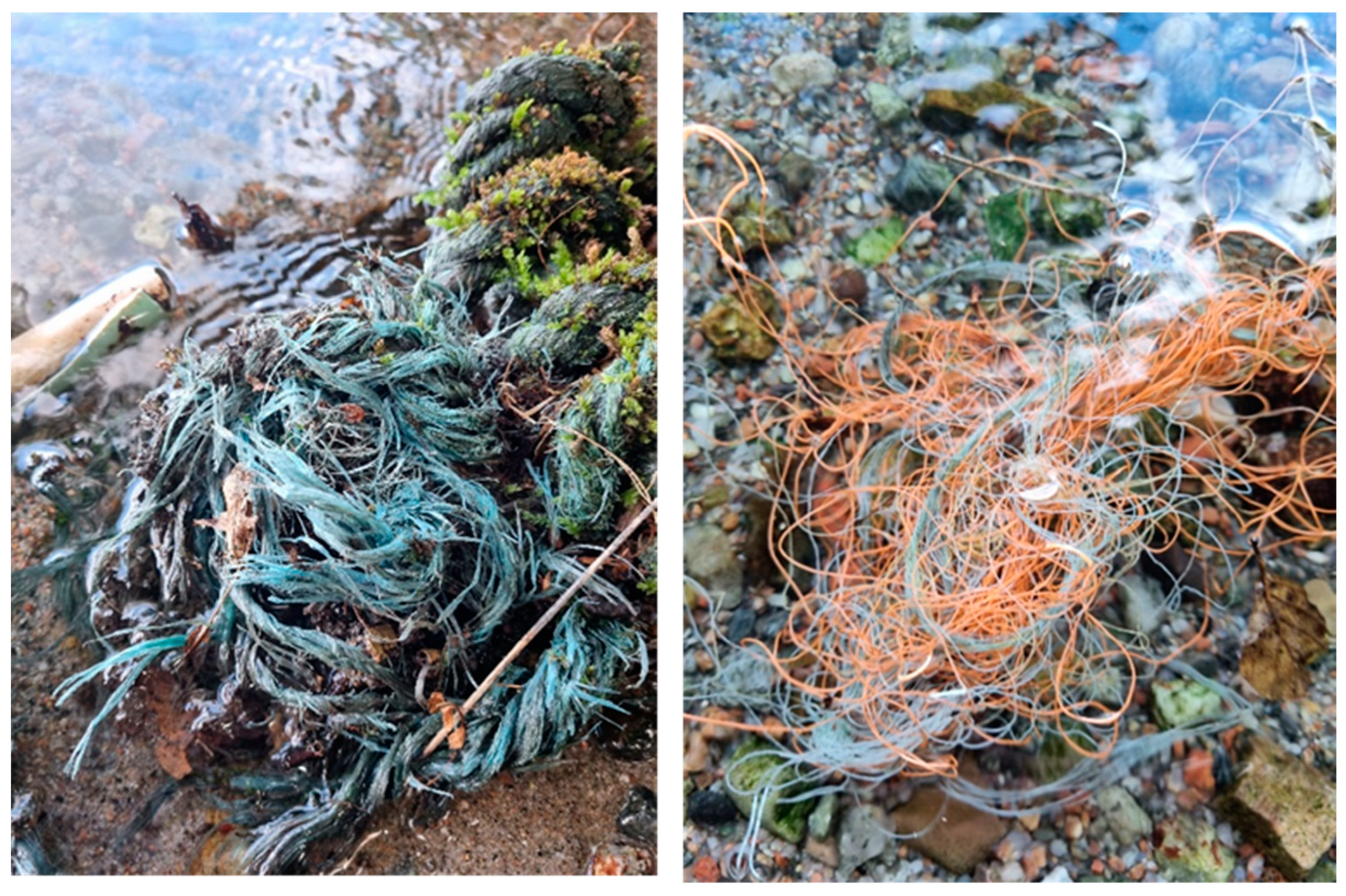The image showcases two panels featuring various pieces of twisted and tangled ropes, strings, or possibly wires washed up on the shores of a body of water, likely a river. The left panel displays a collection of predominantly light blue and greenish twine spread across a brown, rocky ground. Notable details include a white rod-like shape on the center-left and patches of moss in the upper right area, with very little grass visible. The right panel depicts a similar scene but with strings or wires mostly orange in color, interwoven with flecks of green and light blue. Rocks and brownish terrain frame the lower right section, while moss and potential water reflections occupy the upper right. Both panels highlight the chaotic presence of what appears to be human-made litter, likely posing a threat to aquatic life and underscoring the need for environmental cleanup.